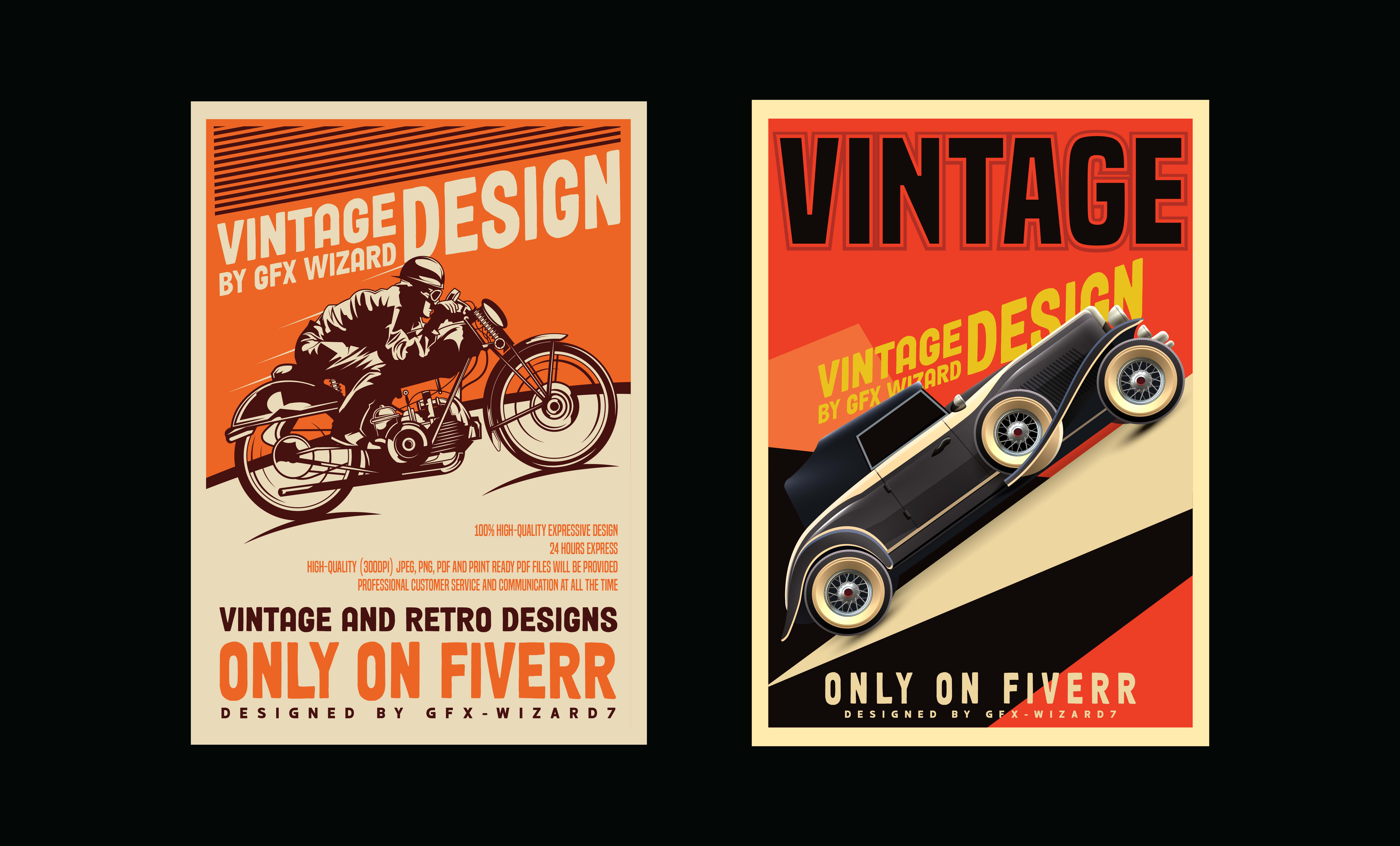The image features a horizontal rectangular black background with two portrait-oriented advertisements centered within it. Both documents share a similar design and layout. 

On the left, there is a vintage-style illustration of a motorcycle with a rider. The motorcycle is depicted in black and white, angled with its front tire pointing to the right and its rear tire slightly lower, giving the impression of an uphill ride. The top of the poster features an orange background with black shading in the corner, and cream-colored text reading "Vintage Design by GFX Wizard." Below this, additional text in orange and black states, "Vintage and Retro Designs" and "Only on Fiber."

On the right, the poster showcases a classic car, likely from the 1950s or 60s, with a luxurious design. The car is dark gray with cream-yellow accents and large white-wall tires, angled with the front facing the top right of the image. The top of this poster has a red background and black text that says "Vintage." The text below, in yellow, reads "Vintage Design by GFX Wizard," and across the bottom in cream text, it states "Only on Fiber."

Together, these posters, set against the solid black backdrop, highlight vintage and retro designs, emphasizing their availability exclusively on Fiber.